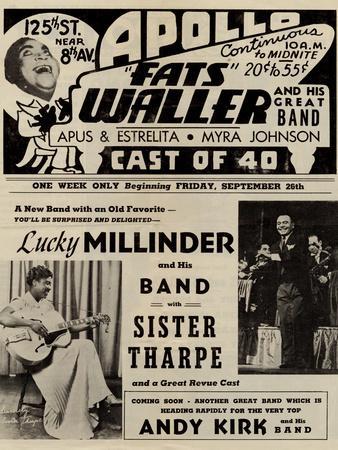This old promotional newspaper clipping showcases an advertisement for the Apollo featuring Fats Waller and his great band. The event boasts continuous performances from 10 a.m. to midnight with ticket prices ranging between 20 cents and 55 cents. Located on 125th Street near 8th Avenue, this one-week-only engagement begins Friday, September 25th. Notably, the ad highlights a new band led by Joaquin Melinder with Sister Tharp, as well as the upcoming performance of another rapidly rising band led by Andy Kirk. Featured prominently are two musicians: a woman in a long white dress playing a guitar, seated, and a man in a tuxedo, smiling, with a microphone, likely onstage. The vibrant text underscores the eclectic mix of talent, including Apus and Estrellita, Myra Johnson, and a cast of 40 performers, promising a spectacular revue.